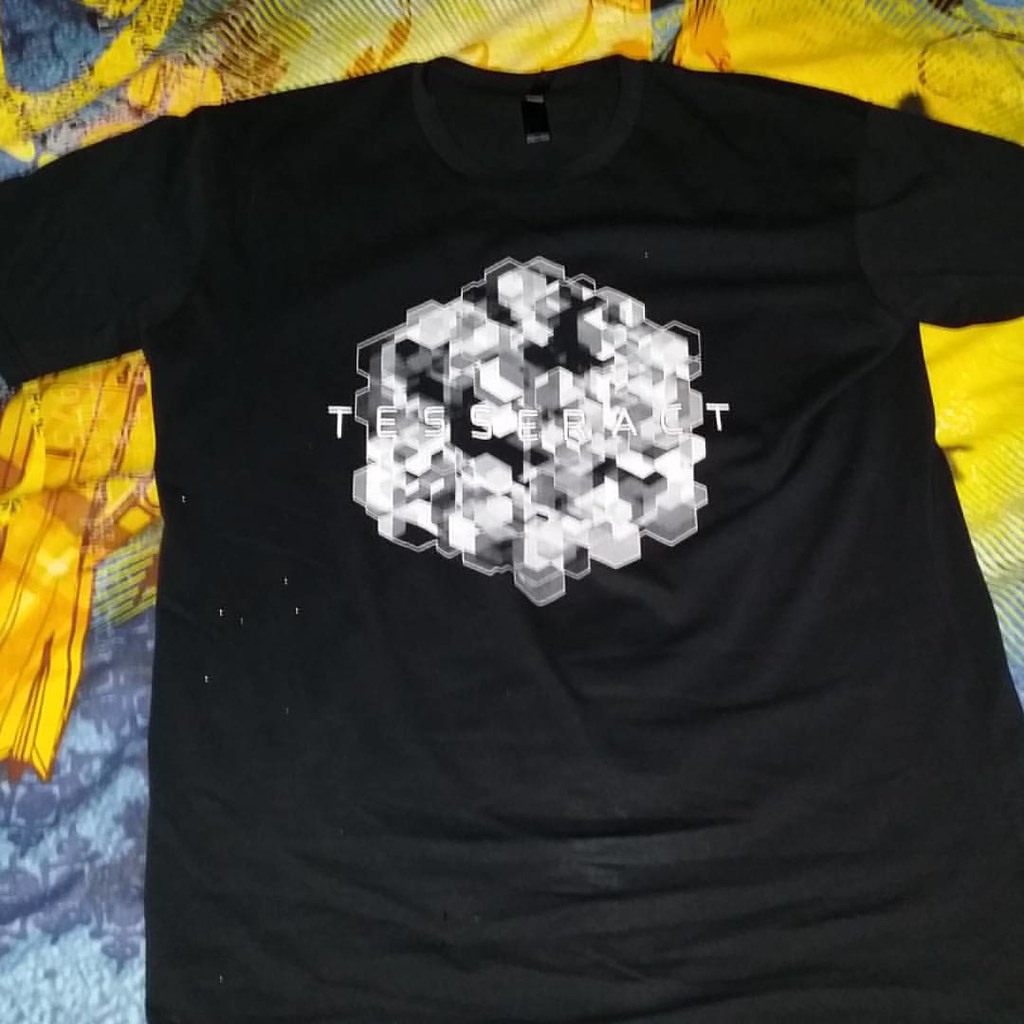A black t-shirt is meticulously placed on a vibrant, colorful painting. The painting, serving as a lively background, features a gradient of colors: a prominent array of blues at the bottom, seamlessly transitioning to golden hues mixed with shades of blue and hints of green as they converge towards the top. Centered on the chest of the black t-shirt is an intricate design of interlocking cubes, collectively forming a larger cube shape. This pattern is rendered in varying shades of gray, white, and black, creating a striking contrast against the dark fabric. Above the cube design, the word "Tesseract" is printed, a nod to the Marvel Universe artifact, albeit depicted in grayscale unlike its famous blue incarnation. The t-shirt appears to be relatively small in size, perfectly accentuating the dynamic artwork beneath it.